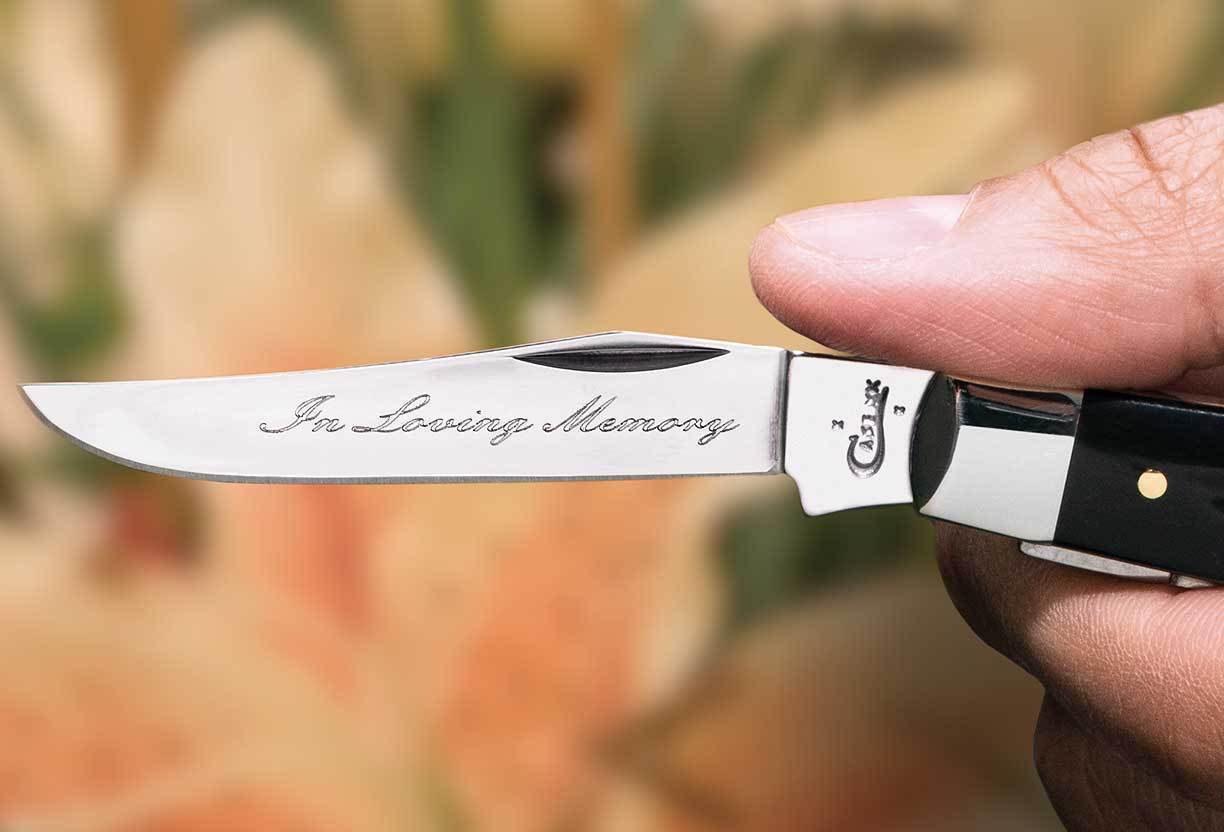This detailed photograph features a pocket knife being held horizontally by a tan-skinned man's thumb and fingers. The knife’s blade, silver with black trim, prominently displays a personalized engraving in script that reads "In Loving Memory." Although mostly clear, some additional numbers and text are partially visible but too difficult to read. The knife’s handle is striking, crafted from black onyx, and includes a distinctive gold dot. The background is softly blurred with variations in white, orange, and green hues, accented with floral patterns, providing a serene backdrop to the sharp, meaningful blade. The positioning of the hand and knife is central to the image, emphasizing the poignant memorial message on the blade.